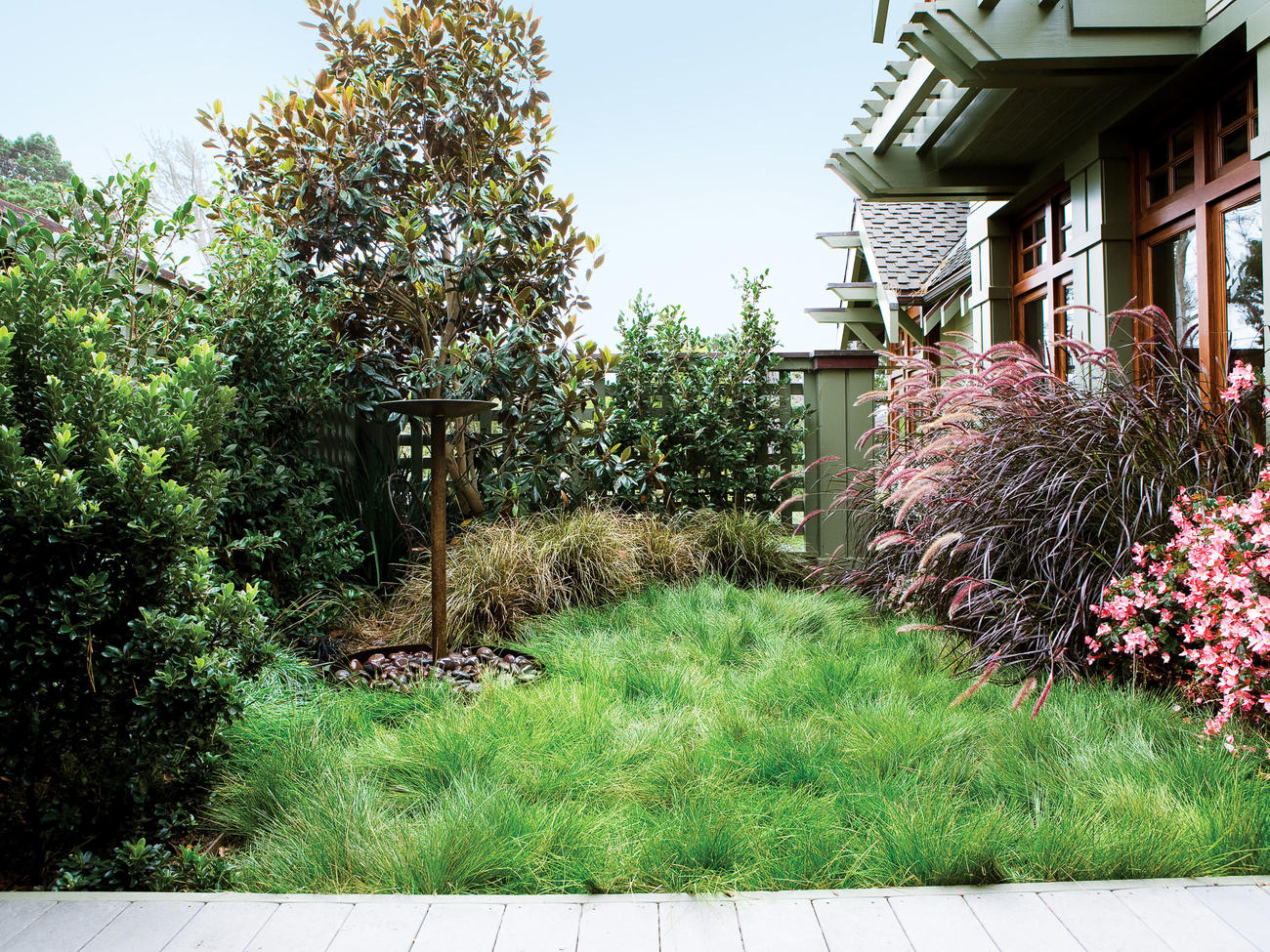This photograph depicts a lush, overgrown yard, most likely part of a residential home's property. Central to the image is a patch of tall, unkempt grass. A wooden walkway runs across the front of the yard, leading eyes toward an ornate wooden house structure on the right side, with light green siding and natural wood-colored windows.

The yard is abundant with plant life. Notably, pink and red flowers are interspersed with vibrant purple and pink plants, including fox tails, adjacent to the house. A wooden fence with lattice-style square openings surrounds the garden, adding to the rustic charm.

Further into the yard, a small tree stands surrounded by a circular mulch bed, flanked by assorted green shrubs and plants. Set beneath this tree is a birdbath or fountain, composed of a circular base filled with rocks, although it appears to be non-operational at the moment. This verdant scene is complemented by additional greenery, including a magnolia tree, that brings a rich diversity of flora to the yard.